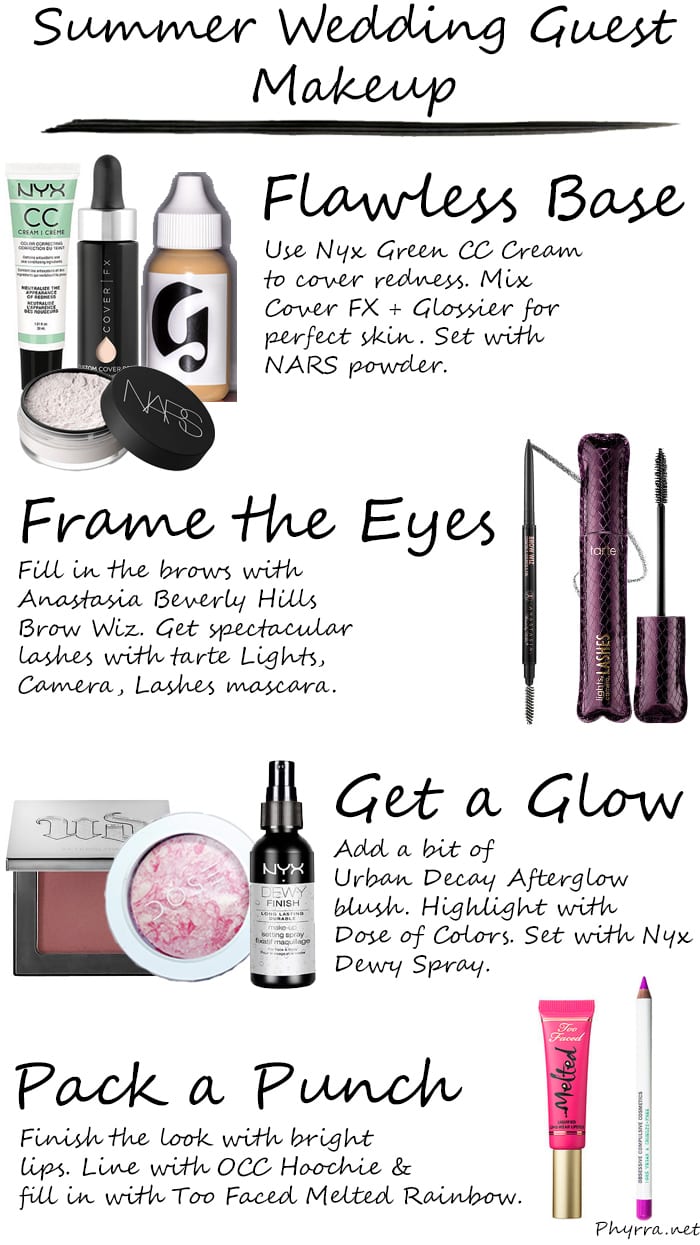### Summer Wedding Guest Makeup by NYX: Your Perfect Look

#### Flawless Base
Create a smooth, even complexion with NYX Green CC Cream to neutralize redness and achieve a flawless base. Various skincare products in elegant tubes and jars contribute to a radiant start for your makeup.

#### Frame the Eyes
Elevate your eye game with precise brushes and eye-enhancing products. Use liners and shadows from NYX to expertly frame and define your eyes, ensuring a captivating look.

#### Glow
Get that summer glow with specialized highlighters and bronzers. This selection of NYX products will help you achieve a luminous, sun-kissed finish.

#### Pack a Punch
Finish off your look with bold, bright lips. Line your lips with OCC Hoochie and fill them in with Too Faced Melted Rainbow for a vibrant pop of color.

#### Brand Overview
This thorough guide features various NYX makeup products designed to help you achieve your perfect summer wedding guest look, ensuring you stand out with elegance and vibrancy.